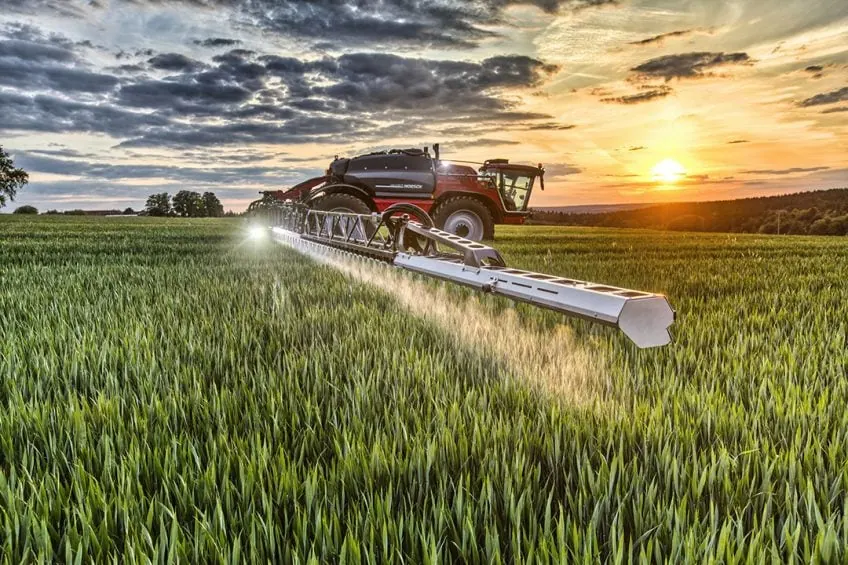The digitally generated illustration depicts a vast farm field with green, grass-like crops. Dominating the scene is a large, red and black tractor-like machine equipped with enormous rubber tires and a glowing headlight at the front. This powerful vehicle features an extensive horizontal panel that sprays water or liquid fertilizer in precise rows over the crops. The backdrop is a sky with a striking contrast: the left side is adorned with dark, wispy clouds against a dark blue backdrop, while the right side is illuminated by a bright, yellowish-orange sun casting a warm glow, suggesting either sunrise or sunset. Trees dot the horizon, adding to the farming ambiance. The scene vividly captures the dynamic interplay between advanced farming machinery and the serene, expansive agricultural landscape.